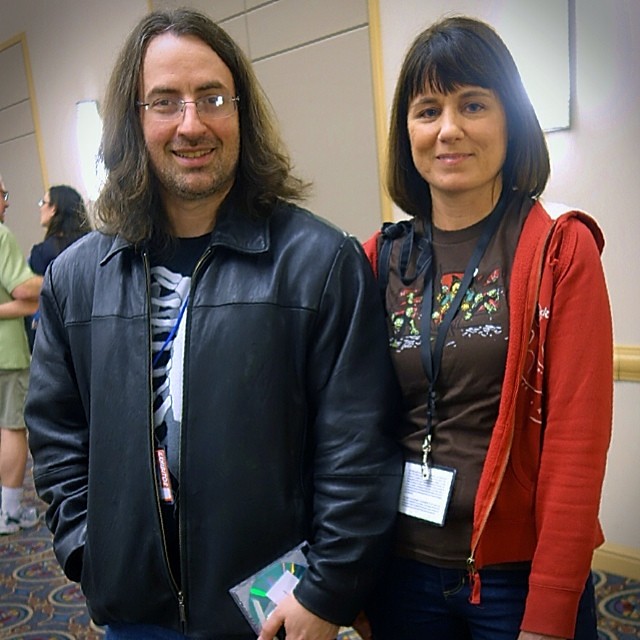In this detailed indoor photograph, two individuals are posing and smiling at the camera. On the left stands a man with shoulder-length, straight brown hair parted to the side, wearing glasses and a subtle smile. He is dressed in a black leather jacket over a black t-shirt featuring a ribcage design. In his left hand, he holds an indistinct object. He appears slightly unshaven, suggesting a couple of days without shaving.

To his right is a woman with shoulder-length dark brown hair styled in a bob with bangs. She is wearing a red zipper sweatshirt over a brown t-shirt that has a colorful design on the chest area. She complements her outfit with dark blue jeans and a black lanyard around her neck, which holds an ID badge with writing visible from the back. She smiles with a closed mouth directly at the camera. The background features a cream-colored wall adorned with white lights, and other people can be faintly observed in the room.